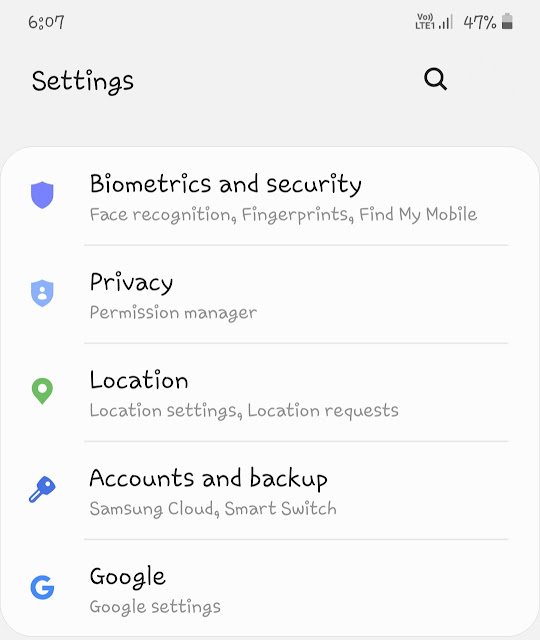The image displays a smartphone screen with various interface elements and settings. 

At the top, there is a light gray status bar. On the top left, the time is displayed as 6:07. On the top right, there are indicators for LTE connection with 3 out of 4 bars, a battery icon showing 47% charge, and other status icons.

Below the status bar, in large black letters, the word "Settings" is prominently displayed beside a magnifying glass icon, indicating a search function.

Underneath, there is a white section with a blue shield icon to the left and the text "Biometrics and Security" to the right. Below this title, it lists options such as "Face Recognition," "Fingerprints," and "Find My Mobile." A light gray horizontal line separates this section from the next.

Further down, there is another section featuring a lighter blue shield icon with a silhouette of a person. This section is labeled "Privacy" and includes options like "Permission Manager." Another light gray horizontal line is beneath this section.

Below the privacy section, a green location pin icon marks the "Location" settings. This area includes options for "Location Settings" and "Location Requests" and is also separated by a light gray line.

Following this, there is a blue key icon next to "Accounts and Backup." Underneath this heading, options such as "Samsung Cloud" and "Smart Switch" are listed.

Finally, another light gray line separates the last section, which features a blue "G" icon next to the word "Google." This section is labeled "Google Settings."